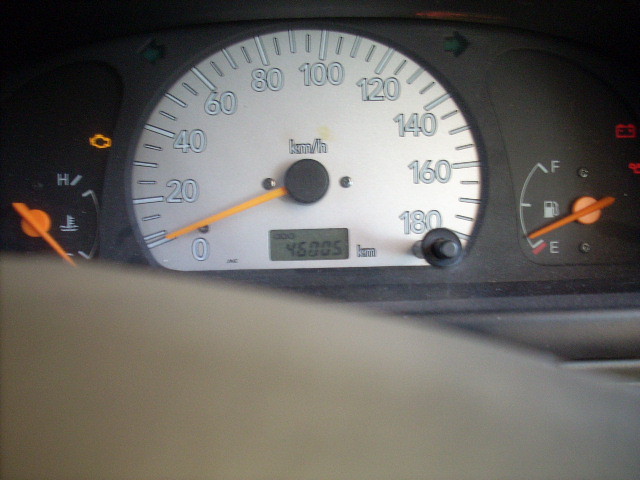This close-up photograph captures the intricate details of a vehicle's dashboard and speedometer gauges. The lower part of the image is blurred by a curved, gray shape—likely the top of the steering wheel—softening the focus in that region. The dashboard itself is a sleek black, creating a stark contrast against the illuminated indicators. 

On the left, the heat gauge prominently features a white line marking the temperature range from 'C' for cold at the bottom to 'H' for hot at the top. A bright orange needle points slightly below the 'C,' indicating a low temperature. Above this gauge, a check engine light is visibly illuminated. 

Dominating the center is a white-backed speedometer, clearly marked from 0 to 180 kilometers per hour. The speedometer's orange needle rests firmly at zero. Beneath the speedometer, a digital readout displays the vehicle's mileage, showing 46,005 kilometers. Nearby, a push button is available for resetting the trip meter. 

To the right, the gas gauge needle hovers just above the empty mark, with a midpoint notch and a line at the top denoting a full tank. Additionally, a red indicator alerts for the battery and oil status, completing the array of critical dashboard information.